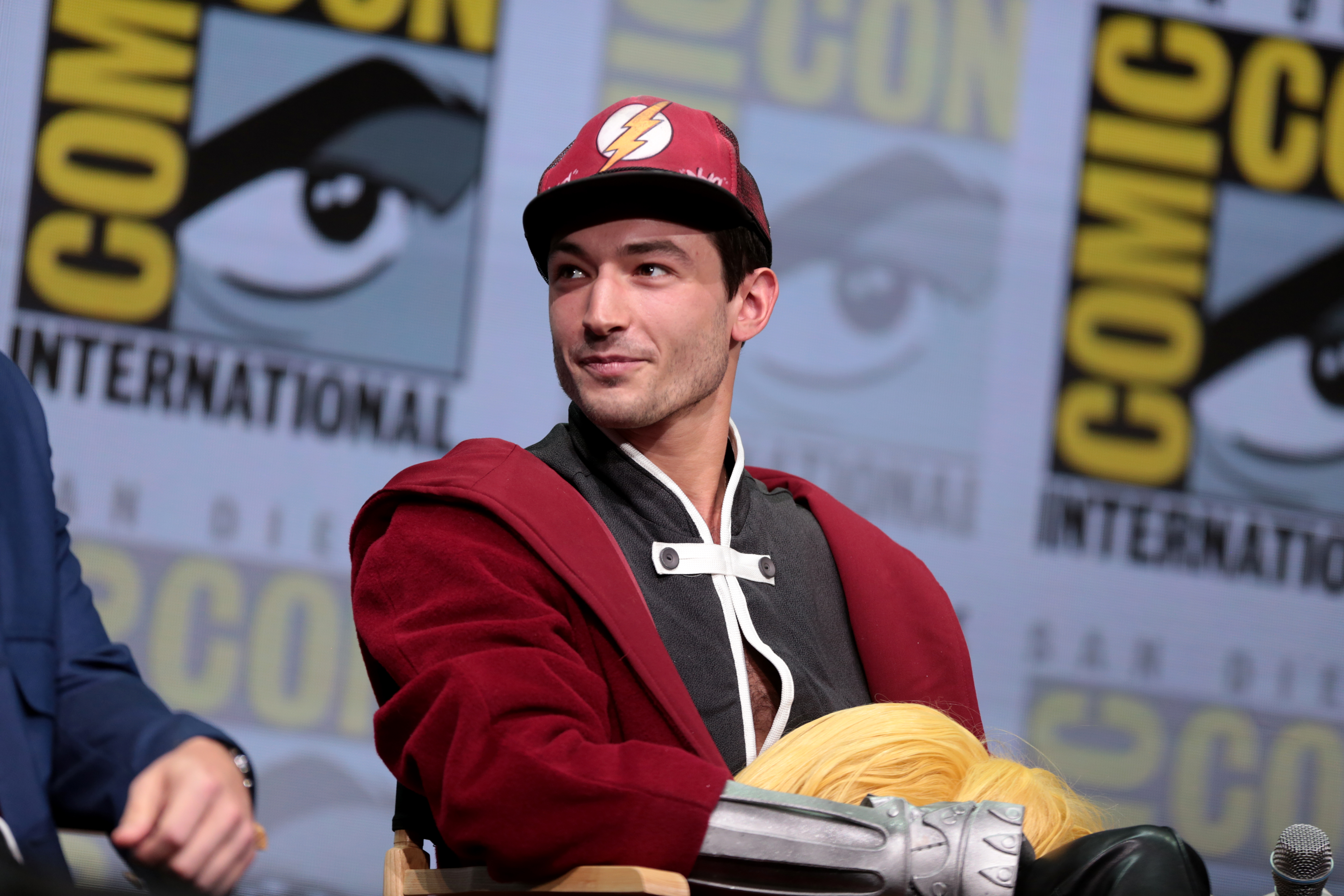This image captures actor Ezra Miller seated at a Comic-Con panel, prominently situated in the center of the scene. Ezra is wearing a striking ensemble: a red jacket layered over a white shirt that features a unique latch just below the neck. Notably, they are also adorned with a gray, plastic gauntlet on their right arm, giving it a mechanical appearance. Their gaze is directed to the left of the frame, towards a fellow panelist donning a red baseball cap emblazoned with the Flash logo, indicative of the character Ezra is known for portraying in DC Comics films. Behind them, the backdrop is repetitively patterned with the Comic-Con logo, featuring the iconic eye and yellow lettering with "International" underneath. A black microphone is visibly positioned in the bottom right corner of the image, likely placed on a table for the panel discussion. Ezra, appearing in their 30s, sports a slight grin, their head angled towards the right in about a seven o'clock position, adding a dynamic element to the photograph.